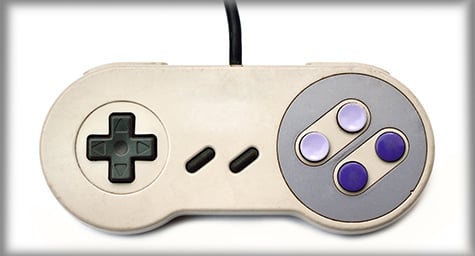The image depicts an older-style video game controller centered on a white background with a shadowy blue gradient border that transitions from darker edges to a lighter middle. The controller, which is predominantly an off-white or light gray color, takes up most of the picture. It has an oblong shape with slightly rounded ends.

On the left side of the controller, there is a black directional pad, often referred to as a D-pad, which resembles an array of up and down arrows. To its right lie two black, pill-shaped buttons arranged in a slant. Moving to the right end of the controller, you will see four circular buttons: two dark blue (or dark purple) and two light blue (or light purple), organized in two smaller slanted, pill-shaped sections. A black cord is attached to the top of the controller, extending upwards and fading out of the picture. The controller appears to be real, possibly photographed on a white surface, and the image is captured from an overhead perspective, displaying an equal horizontal spacing with more room at the top vertically.